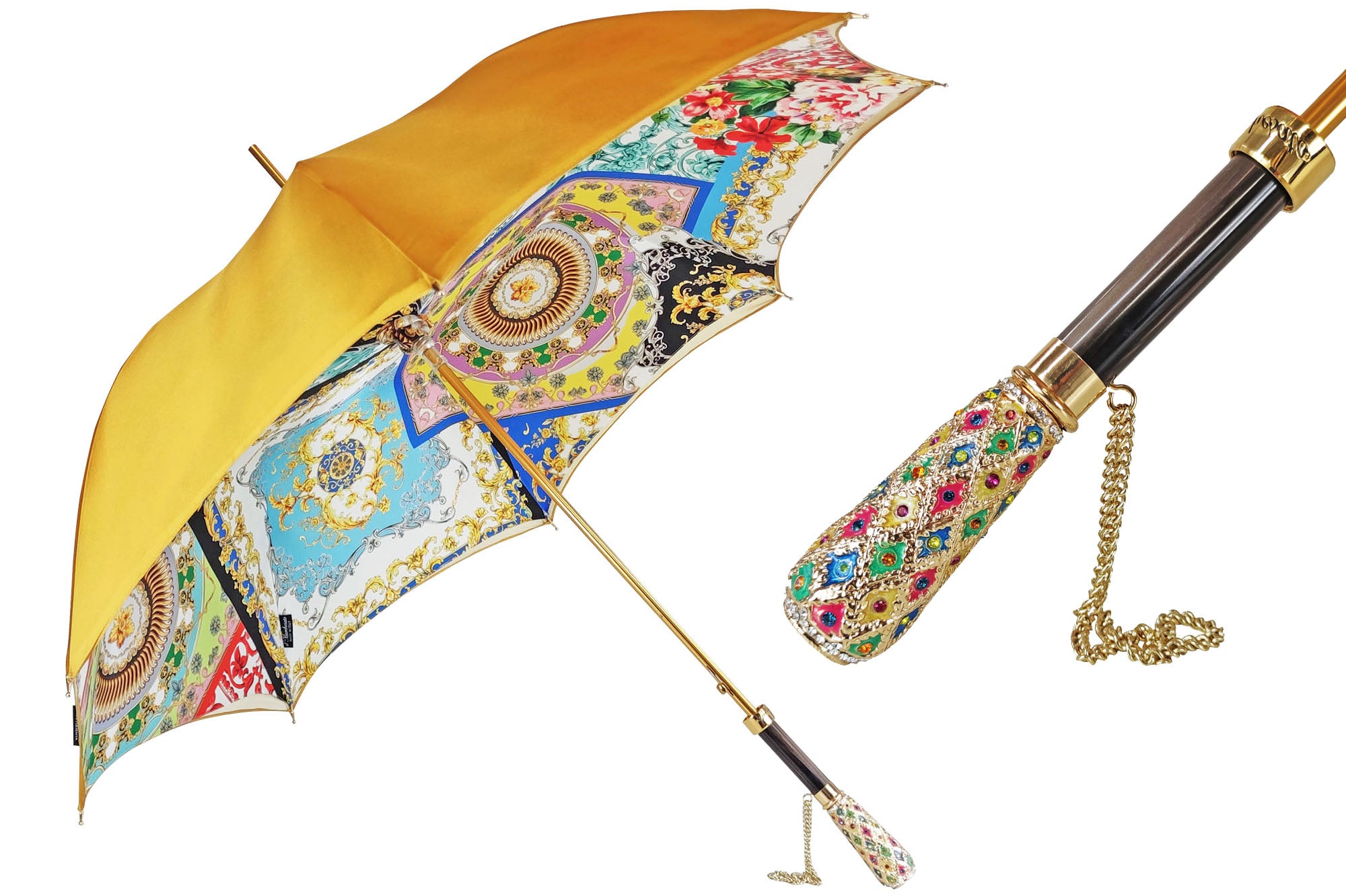The image showcases an artistically elaborate umbrella set against a white background. The umbrella's canopy is a striking yellow on the exterior, while the interior boasts a vibrant array of patterns that include diverse colors and intricate designs reminiscent of paisley prints, circles, squares, and flowers. These patterns feature blue, orange, red, green, and gold fringes, contributing to a rich, ornate appearance. The pole and hardware of the umbrella are gold-toned, enhancing its luxurious feel. The handle, primarily black, culminates in an ornate, jeweled detailing at the bottom, featuring multicolored gems and a pattern of small circular facets. A close-up of this detailed handle is positioned on the right side of the image, highlighting the intricate craftsmanship. The umbrella is presented diagonally towards the upper left corner, open, with the top portion cut out of the frame. This exquisite umbrella also includes a delicate gold chain for holding.